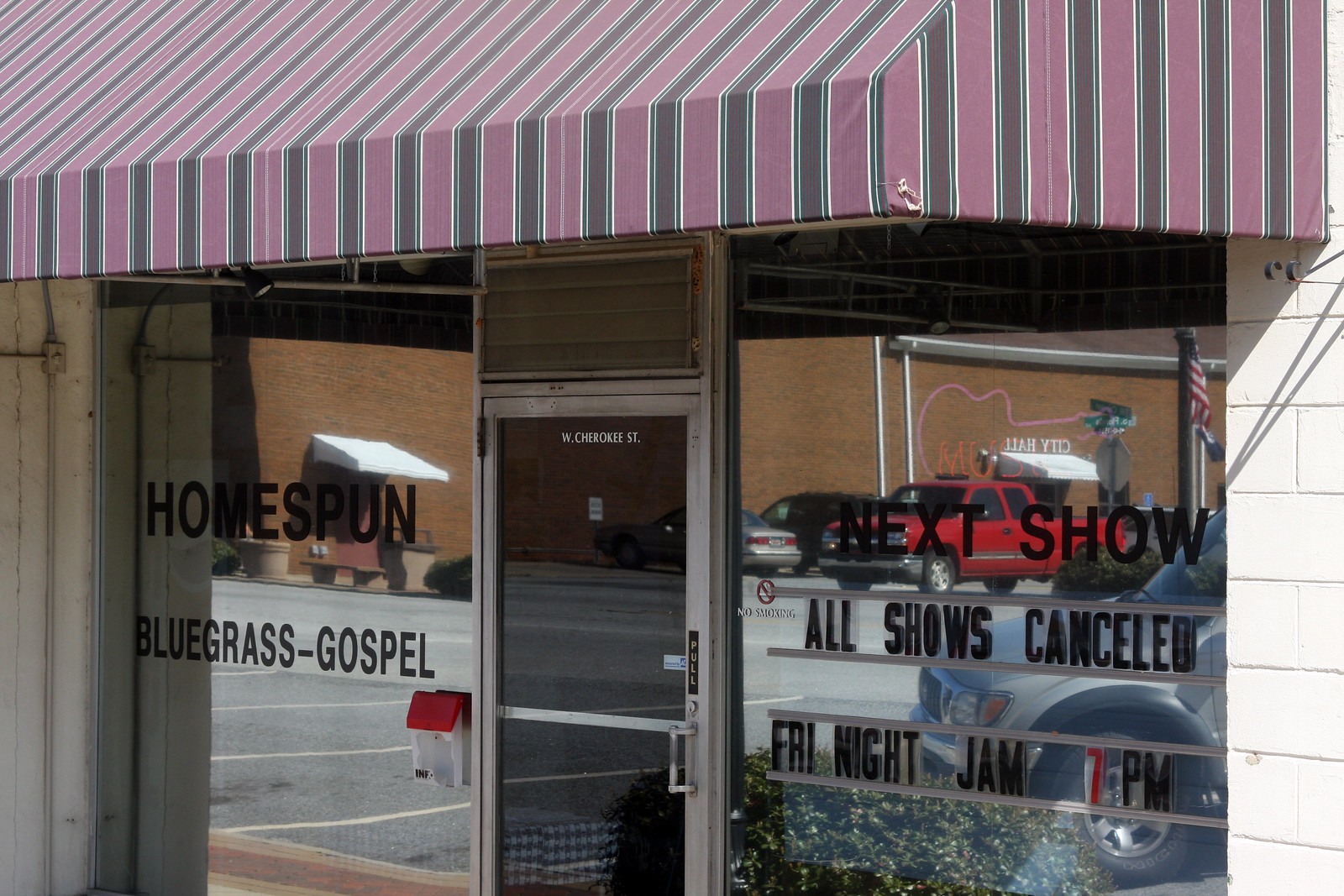The image captures the glass facade of a small music hall, with a centered glass door prominently displaying "West Cherokee Street" in white lettering at the top. To the left of the door, the glass panel is adorned with the text "Homespun Bluegrass-Gospel," while to the right, it announces in white lettering, "Next show, all shows canceled," with "Friday night, jam, 7 p.m." The number "7" is strikingly in red. Stretching across the top of the image is an awning in a distinctive pinkish-lavender shade, featuring vertical stripes in brown and thinner white stripes. Reflections in the glass reveal a red pickup truck and a silver SUV parked in front of the venue, adding a touch of everyday bustle to the scene.